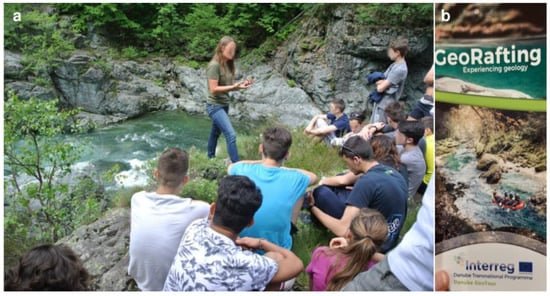This horizontally-oriented color postcard appears to be a promotional advertisement for a georafting company called Inter-Ag. The left side of the image captures a lively outdoor scene set along the serene banks of a river. A woman stands at the center, engaging a group of around 10 to 20 people who are seated in a circle, attentively listening to her. The scene exudes a sense of excitement and anticipation, suggestive of a briefing or orientation for an upcoming adventure.

On the right side of the postcard, a vertical strip features an image of adventurous individuals in a boat, navigating through the river's dynamic waters, encapsulating the thrilling experience of georafting. This strip is adorned with bold, white text at the top that reads "GEORAFTING," along with the company's logo, "Inter-Ag," displayed at the bottom. A thin white border neatly separates the vibrant outdoor scene from the energetic boating image, maintaining a clear distinction between the two visual elements.

Overall, the image cohesively showcases the adventure and camaraderie of georafting, enticing potential vacationers to explore this exciting activity with Inter-Ag.